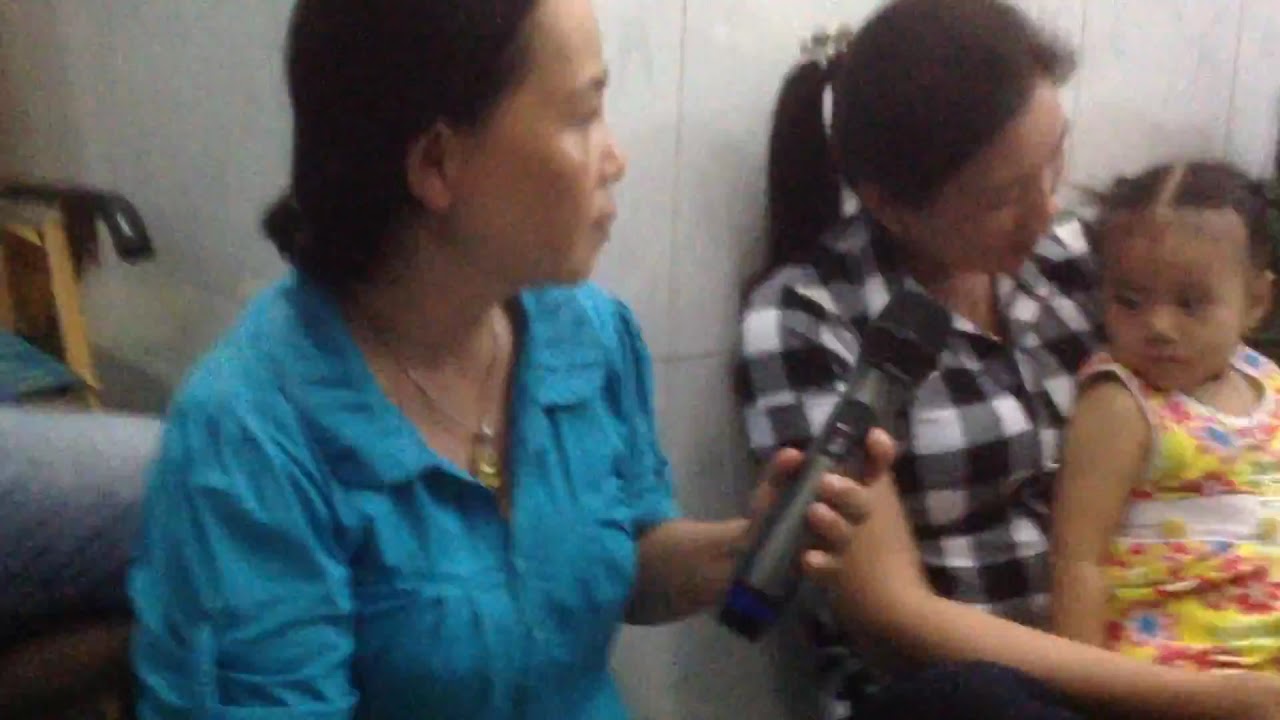This photograph captures a detailed scene of two Asian women sitting indoors against a white wall backdrop. The woman on the left wears a turquoise-blue top with a collar and a gold chain necklace featuring a hoop pendant. She has short, jet-black hair combed back and holds a black microphone with a gray body and black head in her left hand. She is looking to her left, towards another woman and a child. 

The woman on the right is dressed in a short-sleeved black and white checkered shirt and has her black hair tied up in a ponytail. She holds a little girl on her lap. The child, who appears to have her hair tied up in two knots and parted in the middle, is wearing a vibrant yellow dress with a blue and red floral pattern. The child is looking at the microphone, seemingly curious but not reaching for it. Behind the women, there is discernible seating furniture, adding context to the indoor setting.